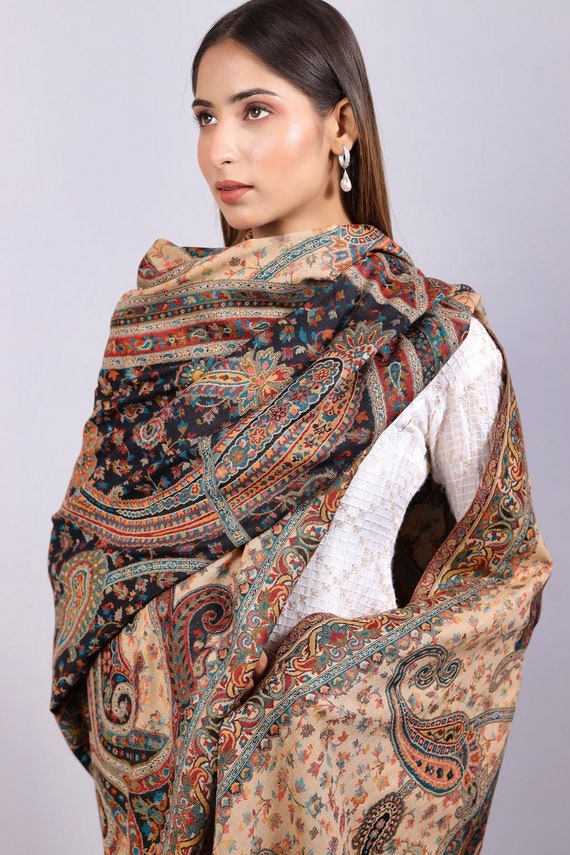The image features a female model of Indian descent with medium tan skin and long, straight dark brown hair that extends halfway down her back. She is standing slightly angled away from the camera, presenting a three-quarter view. The model wears an Indian-style ensemble, including a long, loose-fitting wrap that begins around her neck and drapes down her body, partially exposing a white, slightly rough-textured garment underneath adorned with gold, crisscrossing diagonal embroidery.

The wrap is likely made of silk and showcases an intricate paisley pattern in a rich palette of tans, reds, golds, blues, and turquoise. The wrap is held in place by the model's left hand, and her left ear is visible, adorned with large, diamond-encrusted earrings that add a touch of elegance to her look. She stands against an abstract gray background, creating a striking contrast that highlights the intricate details of her attire and accessories.